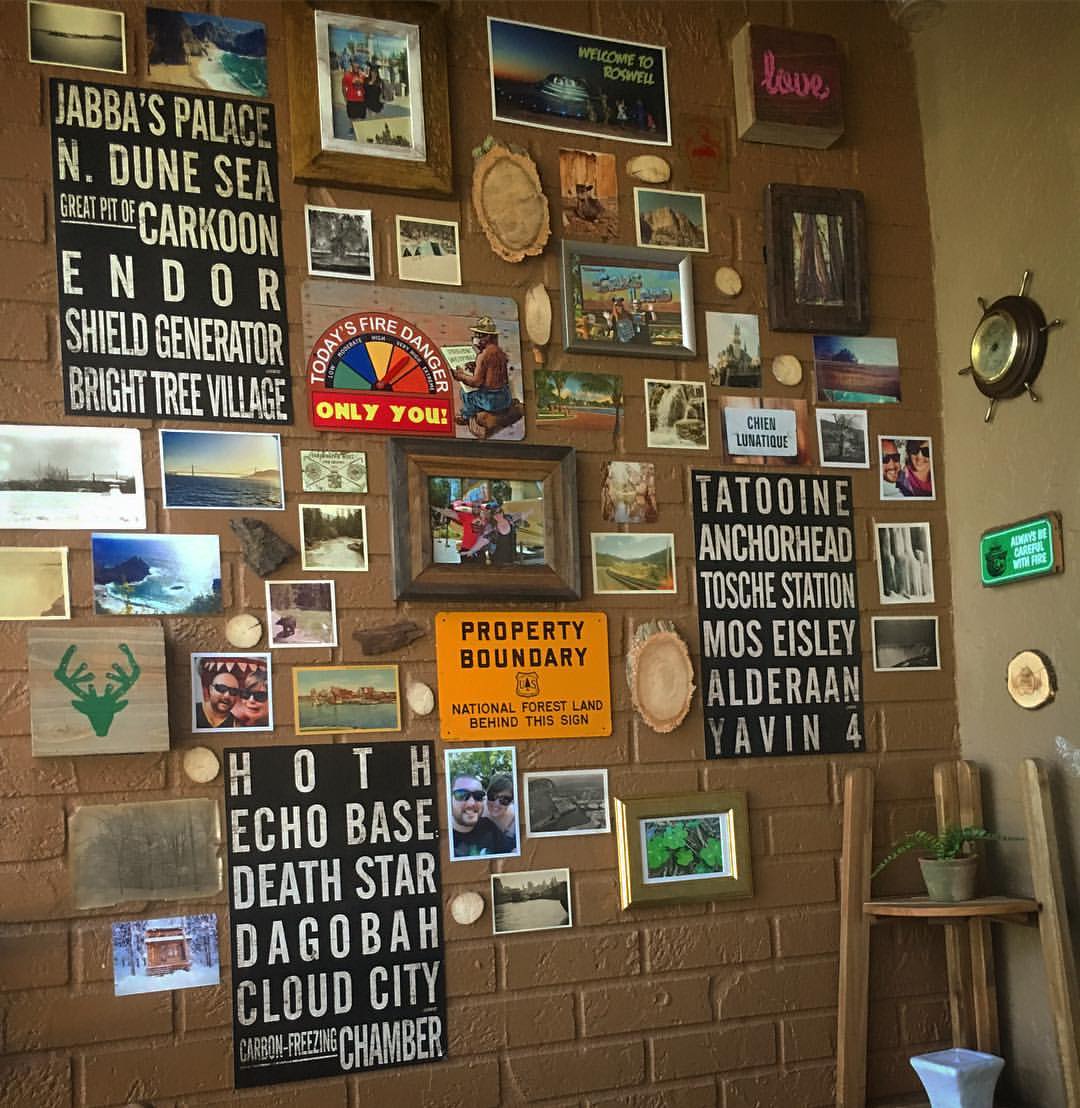The photograph captures a detailed view of an eclectic, decorated corner inside a room, where the primary focus is a dark brown painted brick wall adorned with a diverse assortment of posters, pictures, and souvenirs. At the top, there are photographs of beaches viewed from different angles, accompanied by additional beach images and a snapshot of Disney World visitors. Significantly, a large black poster lists destinations like Jabba's Palace, North Dune Sea, Great Pit of Carcoon, Endor, Shield Generator, and Bright Tree Village. A vibrant graphic sticker next to it indicates "Today's Fire Danger," with an adjustable red arm and a bear in blue jeans and a ranger's hat on a log, emphasizing "Only You."

Moving downwards and to the right, a postcard shows a UFO scene and welcomes viewers to Roswell. Within the collage of images is also included a photograph of tents on a beach. A notable wooden stool with a potted plant sits to the left corner of the wall. The adjoining plain wall features wall hangings including a clock and an empty white vase on the floor. 

Notably absent among the captured items are smaller detailed posters, one reading "Property Boundary, National Forest Land," underscored with a logo, and another (possibly fictional) listing locations such as Hoth Eco Base and other places from the Star Wars universe. A "LOVE" wall hanging further adds to the mélange of items. Together, these elements create a visually busy and richly decorated wall, narrating a story through travel, nature, fictional, and nostalgic themes.